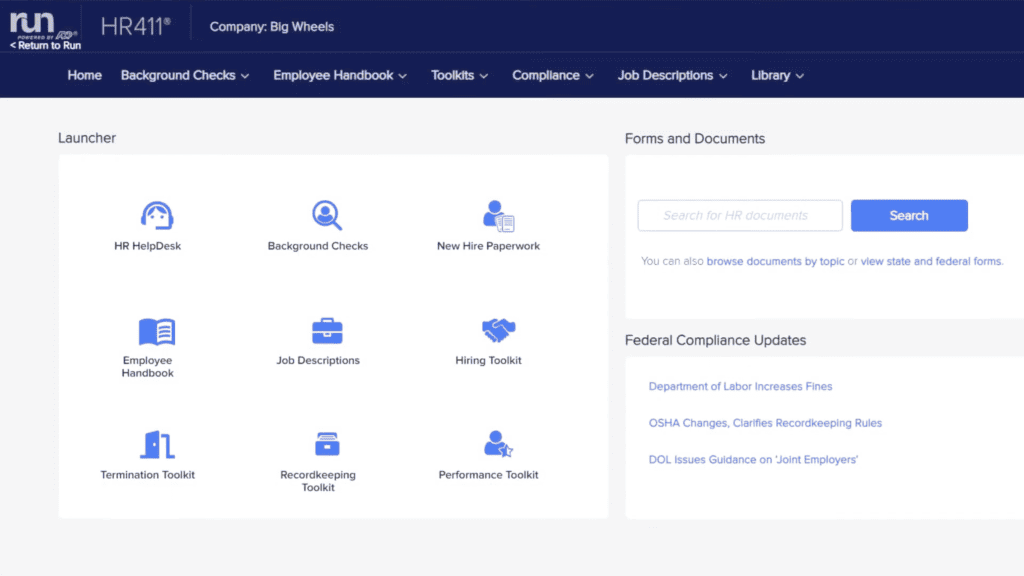The image showcases a software interface called "RUN," spelled out clearly as R-U-N, with the heading "Return to RUN." Prominently featured is a bright arrow pointing towards the main title. Below the header, various company-related sections are displayed, including "Home," "Background Checks," "Employee Handbook," "Toolkits," "Compliance," "Job Descriptions," and "Library," each accompanied by dropdown menus for further exploration.

At the top, the headings appear in black with white lettering. The subsequent section features a gray box labeled "Launcher" in black text, with a white box containing various icons and descriptions. Each icon represents different tools:

- **Help Desk**: Icon of a person with a microphone.
- **Background Checks**: Icon resembling a private investigator.
- **New Hire Paperwork**: Blue icon of a person with documents.
- **Employee Handbook**: Icon of an open handbook.
- **Job Descriptions**: Icon resembling a small suitcase.
- **Hiring Toolkit**: Icon of a tiny toolkit.
- **Termination Toolkit**: Another toolkit icon.
- **Records Keeping Toolkit**: Icon resembling a safe box.
- **Performance Toolkit**: Icon of a person.

On the right side of the interface, there is a section titled "Forms and Documents," which includes a search bar for easy navigation. Additionally, several compliance updates are listed, such as "Federal Compliance Update," "Department of Labor Increases Fines," "OSHA Changes and Clarifies Bookkeeping Rules," and "DOL Issues Guidance on Joint Employers."

This interface serves as a comprehensive launcher program to help users navigate and access various company resources efficiently.